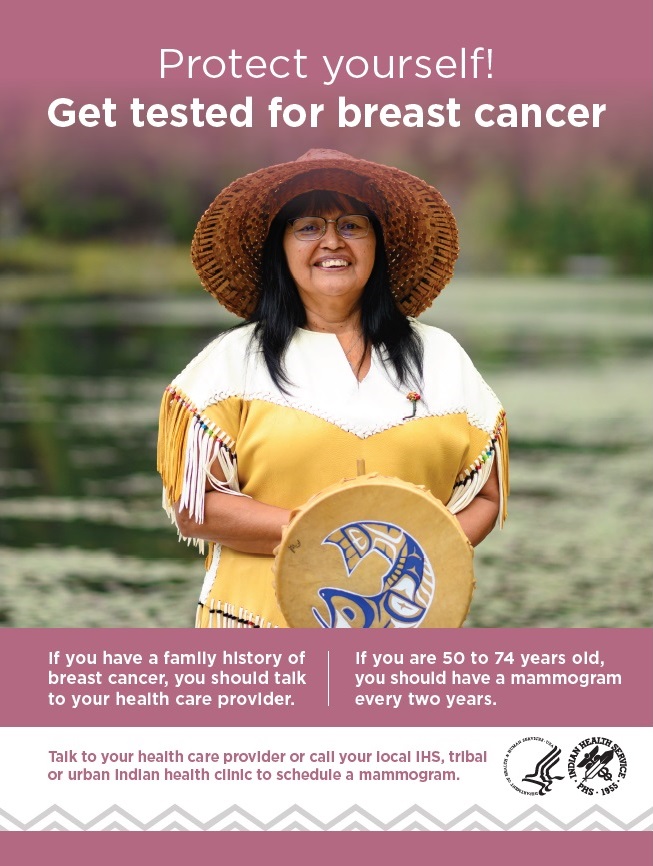This is a rectangular, pink-bordered advertisement from the Indian Health Services (IHS), primarily aimed at Native American women. The prominent headline at the top, in white font, reads, "Protect Yourself, Get Tested for Breast Cancer." Below this message is a photograph of a middle-aged Native American woman. She is smiling warmly, wearing large black glasses, and a wide-brimmed straw hat. Her long black hair cascades down, and she is dressed in a yellow shirt adorned with a white collar and yellow and white fringe on the sleeves. She holds a drum featuring a blue and white fish design.

The poster's text continues below her image, offering critical health advice: "If you have a family history of breast cancer, you should talk to your healthcare provider. If you are 50 to 74 years old, you should have a mammogram every two years." A white banner with pink lettering at the bottom instructs, "Talk to your healthcare provider or call your local IHS tribal or urban Indian health clinic to schedule a mammogram." It also includes the IHS logo and a gray triangle pattern as part of the design. This visually engaging poster is likely meant for display in medical settings such as doctors' offices or gynecology clinics, with the goal of encouraging timely breast cancer screenings.